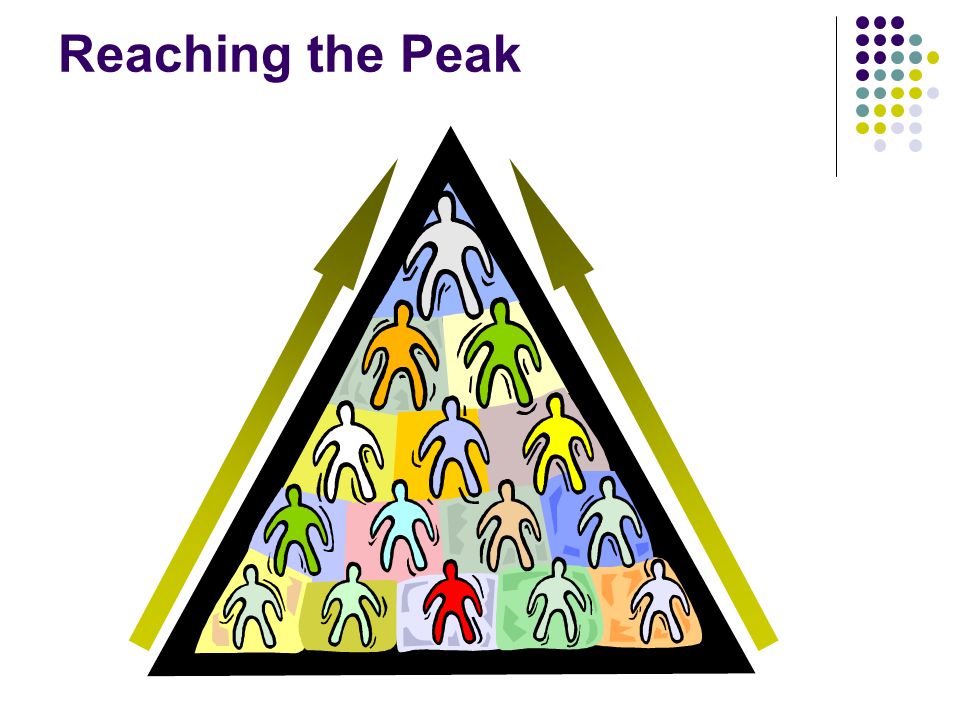This striking computer art image features a white background with a central black-bordered triangle. Inside the triangle, human figures of various colors—white, yellow, green, orange, blue, and red—are arranged from the base, where they are numerous, to the apex, which holds a single figure, illustrating an ascent towards a goal. The top left corner of the image displays the motivational phrase “Reaching the Peak” in purple text. Complementing this are two arrows on either side of the triangle, both pointing upwards, symbolizing progress and ambition. To the top right, an intricate design of multicolored dots forms a logo or emblem. This pattern consists of vertical columns of dots in shades of purple, blue, yellow, and gray, separated by a vertical black line, adding a structured aesthetic to the dynamic composition.